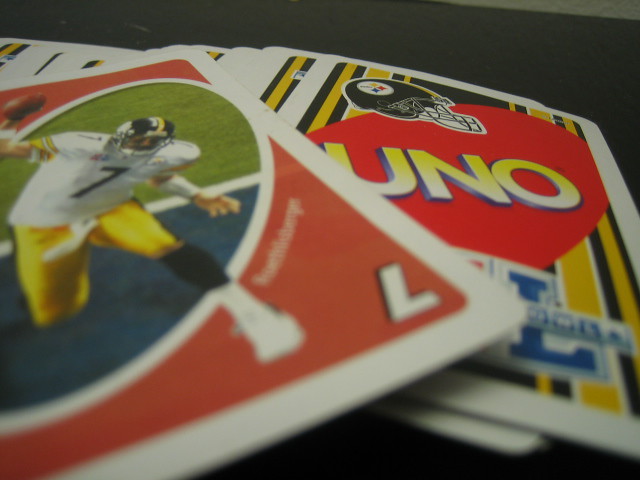In this image, we see a collection of football-themed UNO playing cards scattered on a black tabletop. The majority of the cards are face down, fanned out from left to right, as if pushed over from an initial stack on the left. Each card features a prominent red oval shape in the center with the word "UNO" in bold yellow and white uppercase font, accented with a gray shadow. Above this text is a black football helmet with its face guard pointing to the right, adorned with a white circle logo containing three colored diamonds—yellow at the top, red to the right, and blue at the bottom—reminiscent of a football team insignia. The background of these cards features vertical yellow and black stripes, bordered in white.

Dominating the left half of the frame is a single card flipped face up. This card boasts a vibrant red background with a similar diagonal oval shape, displaying a photograph of a football player. The player, wearing a black helmet and a white jersey with the number seven prominently displayed on his chest, also sports yellow pants, black knee-high socks, and white shoes. He is captured in mid-action, holding a football above his head with his left hand while running forward. The ground beneath him is artistically shown with a blue section at the bottom, followed by a white line, and finally green grass. The number seven is also located in the lower right corner of this card.